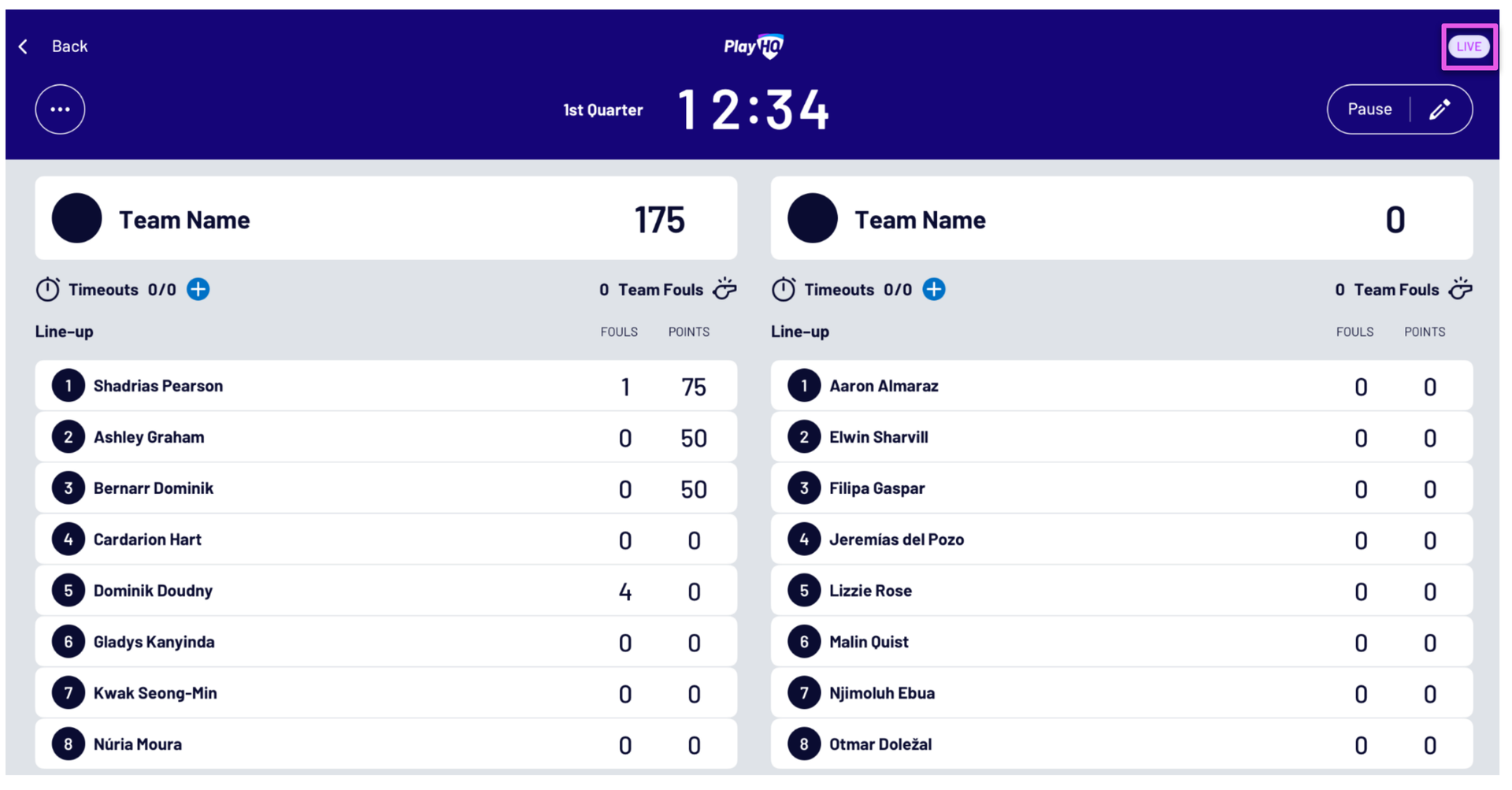The image displays a single screen segmented into various informational sections, heavily focused on a live sports game interface. At the top, there's a thick blue band featuring white text. On the left side of this band, "Back" is written, while the center reads "Play HQ." Directly underneath this center text, it says "First Quarter" followed by the time "12:34." Towards the right, there is a "Live" indicator enclosed in a purple-pink box.

Below this header, additional information is segmented. On the left, it displays "Team Name" with a score of "175" on the right. Details underneath include "Timeouts: 0/0," a plus sign (+), and "0 Team Fouls." The lineup comprises eight players:
1. Shiraris Peterson: 1 foul, 75 points
2. Ashley Graham: 0 fouls, 50 points
3. Bernard Dominic: 0 fouls, 50 points
4. Cardion Hart: 0 fouls, 0 points
5. Dominic Downley: 4 fouls, 0 points
6. Gladys Kendi: 0 fouls, 0 points
7. Kiswak Seagong Ming: 0 fouls, 0 points
8. Nuri Moura: 0 fouls, 0 points

On the opposite side, the screen mirrors the structure: "Team Name" is displayed with a team score of "0" to the right and "Timeout: 0" below it. The bottom part of the screen includes additional controls labeled "Pause" and "Edit."